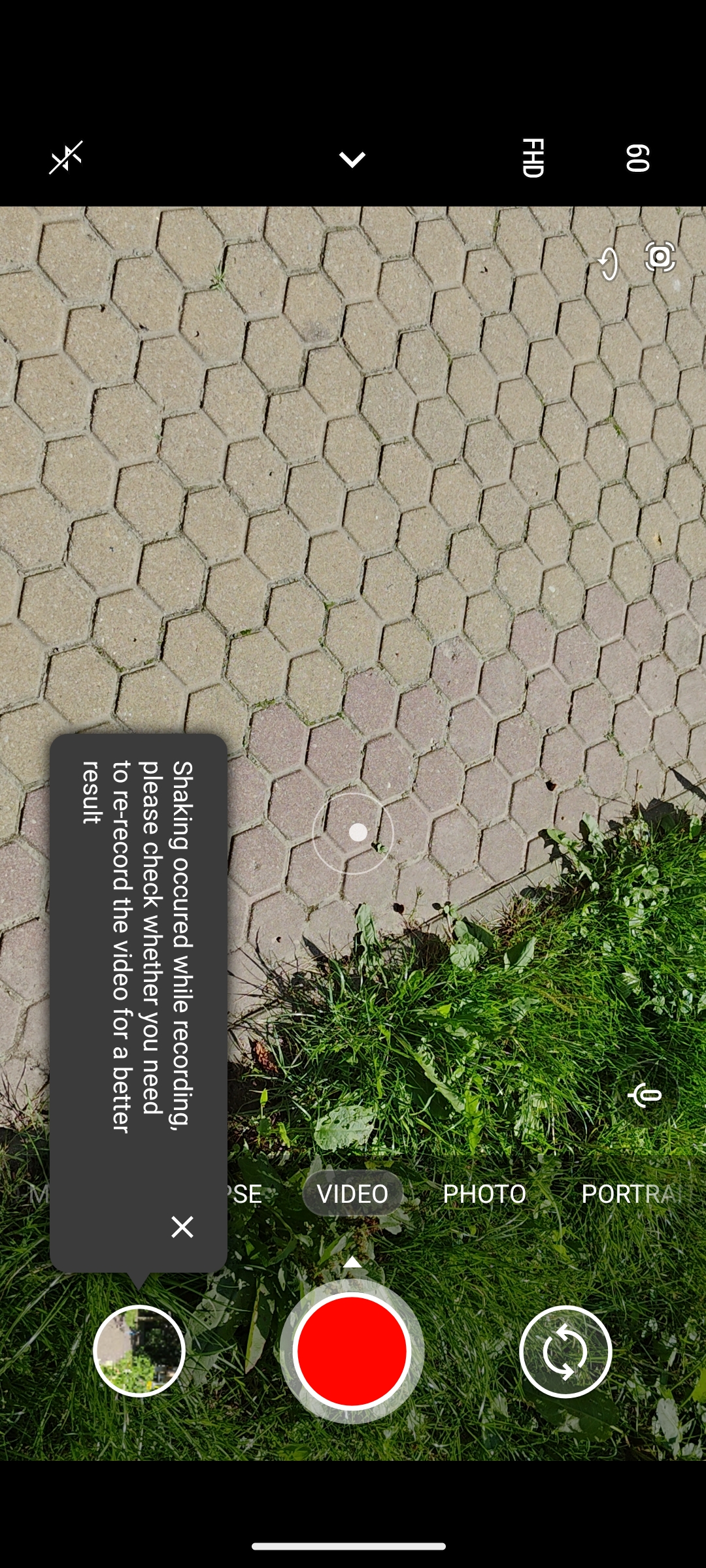The image is a screenshot taken from a smartphone. At the top of the screen, there are several small icons, although their specific details are not clear. Dominating the middle of the screen is a downward-pointing arrow icon. The phone's background features a photograph of a wall adorned with light gray hexagonal shapes arranged side by side. This wall is positioned against a backdrop of a green lawn that appears poorly maintained, with a mix of lawn grass and weeds.

On the left side of the screenshot, a gray rectangular text box is oriented vertically, requiring a 90-degree turn to read it properly. The white text within this box reads: "Shaking occurred while recording. Please check whether you need to re-record the video for a better result." A small 'X' in the upper right corner of this box allows the user to close the message.

At the bottom of the screen, there are several selectable options for different modes. Although the text box obscures two of them, the visible options are, from left to right: "Video," "Photo," and "Portrait."